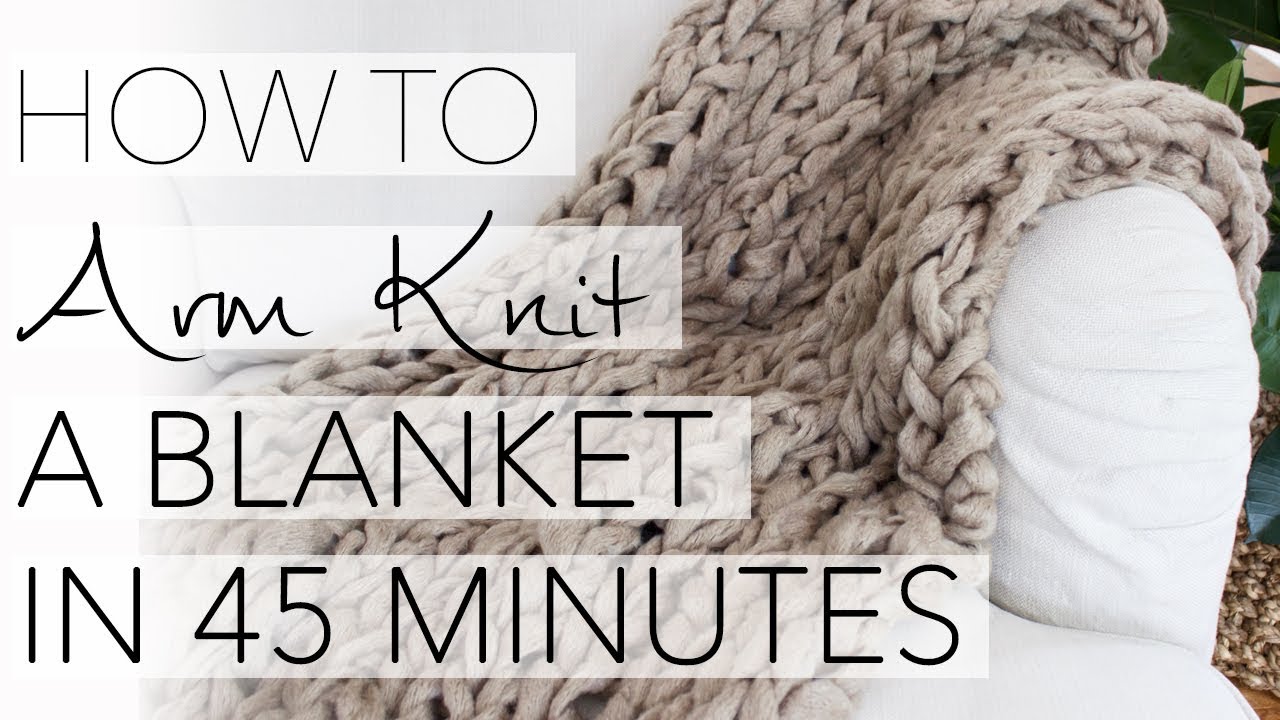The image is a screenshot of a video that demonstrates how to arm knit a blanket in 45 minutes, with a bold text overlay stating, "How to arm knit a blanket in 45 minutes." The blanket, which is prominently featured in the scene, is a sandy brown, light beige color with large, loose cable knits. It is draped in soft folds over the edge of a white fabric-covered sofa. In the background, a tan or khaki braided rug can be seen on the floor next to the sofa, while the leaves of a plant peek in from the top right corner, adding a touch of greenery to the cozy setting. The overall composition suggests an arts and crafts tutorial, possibly serving as a thumbnail for a YouTube video.